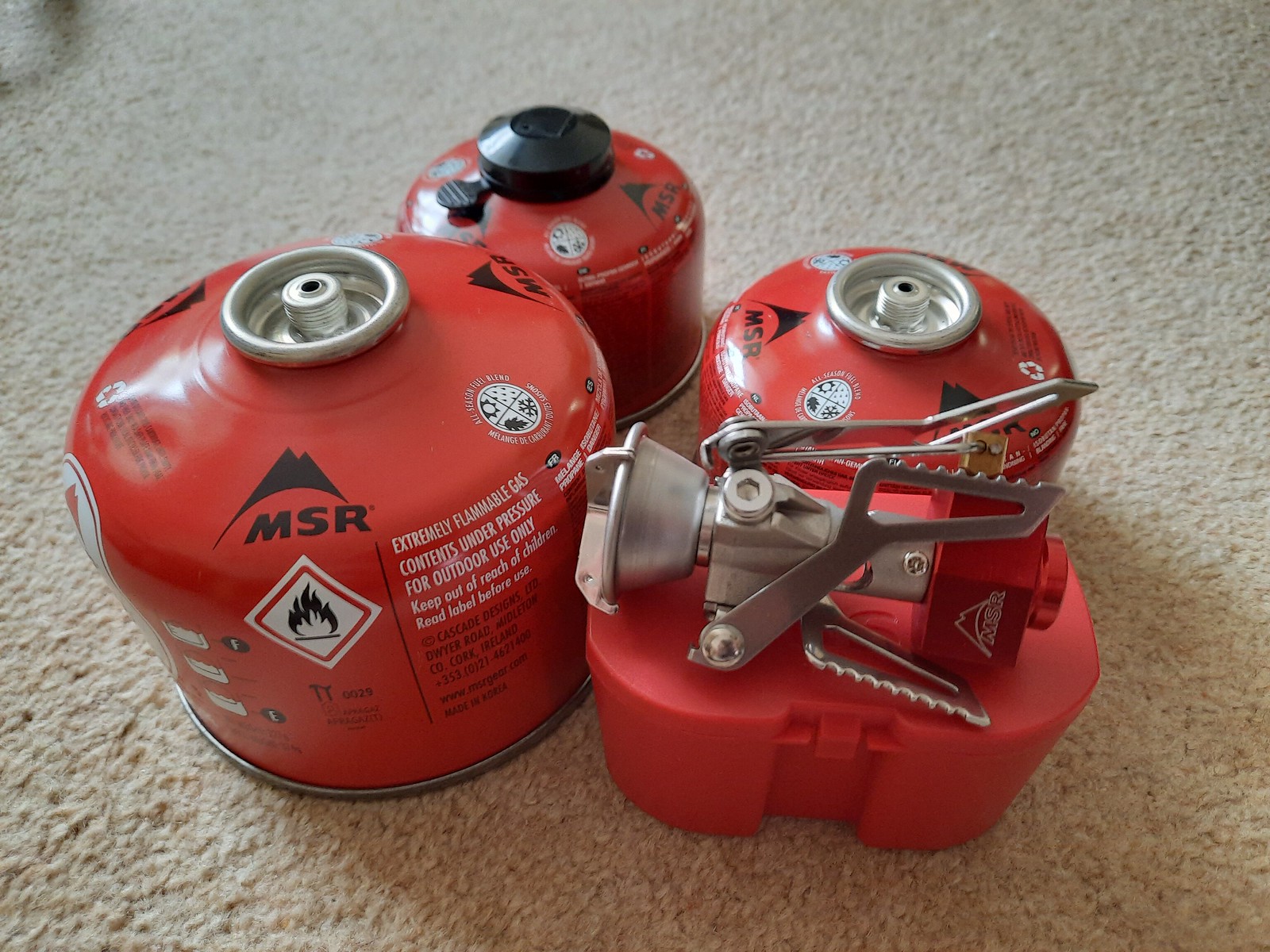The image is a detailed close-up color photograph taken from above with a flash. At the center, there are three red cylindrical fuel canisters of varying sizes, each with a metal top and screw, bearing a warning and a fire logo indicating they are extremely flammable. They are arranged on a well-worn, beige carpet that appears to have been trodden on multiple times. In addition to the canisters, there is a red plastic case positioned to the right-hand side. Resting atop this case is a metal camping gas single burner cooker, identifiable by its jagged edges and silver finish. The setup, which seems designed for showcasing the items for sale on an online marketplace like eBay or Gumtree, suggests a practical camping ensemble ready for use.